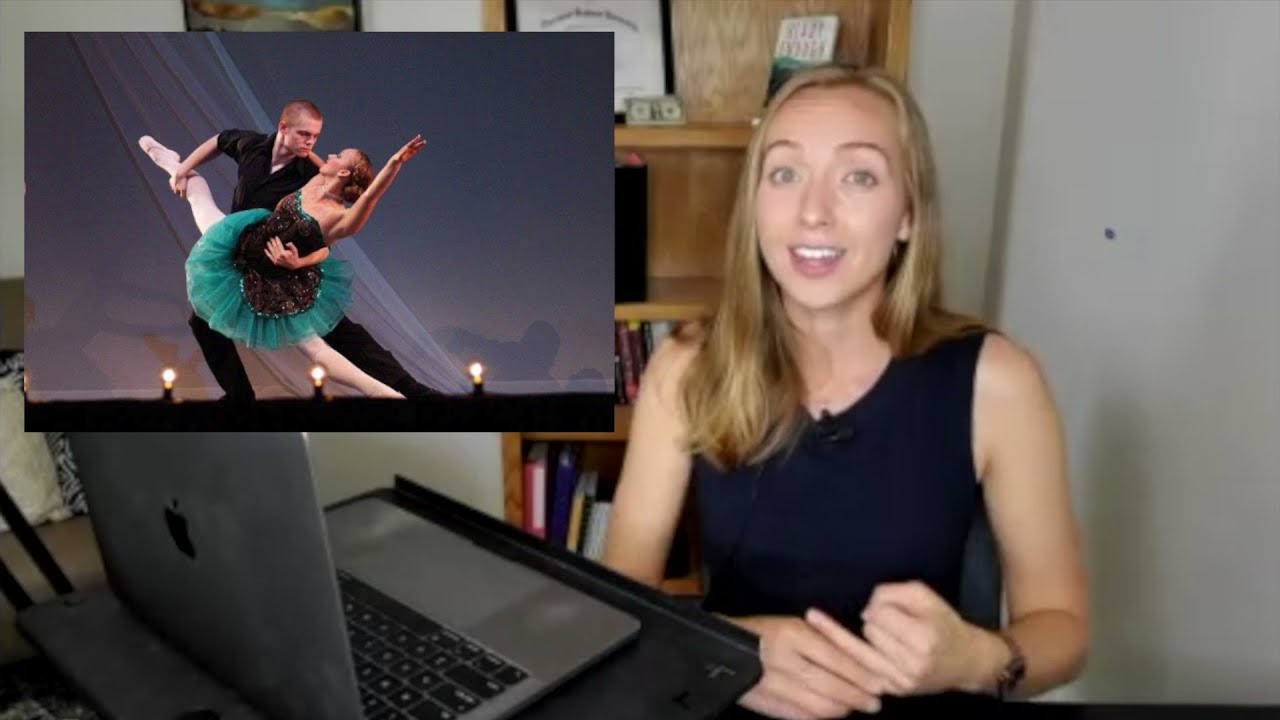The photograph appears to be a screenshot from a blog, showcasing a woman in an office setting. She is seated at a desk with a silver MacBook on a black stand in front of her. The woman, who is white with long, blonde hair and wearing a sleeveless navy-blue top, also has a black lapel microphone clipped to her blouse. Her hands are clasped together, and she's gazing intently at her laptop, seemingly reacting to or explaining something.

Behind her, there is an off-white drywall with a light wooden shelf holding various books and a framed diploma positioned on the top left-hand side. In the upper left-hand corner of the image itself, there is a rectangular cutout depicting two professional dancers on a stage. In this dance scene, a white male dancer with thin blonde hair and dressed in black is holding a female dancer by the waist and raising her left leg. The female dancer is wearing a dark burgundy and green tutu, and she has blonde hair with her left arm extended out. The woman in the main photo has a wide-open mouth, showing her pink lips and white teeth, indicating she might be reacting with surprise or enthusiasm to the dance performance displayed.